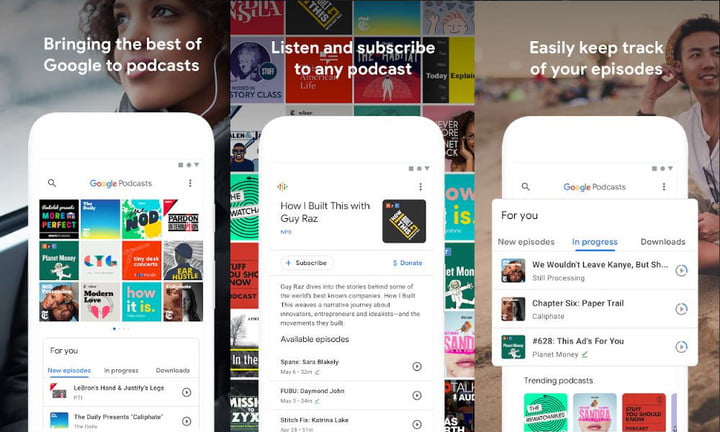This screenshot features three promotional images highlighting Google Podcasts. Each image emphasizes different functions and the user-friendly interface of the app. 

**Left Image:**
An African American woman is the main focus, with the text "Bringing the best of Google to podcasts" overlaying the top part of the photo. Below her, a phone screen showcases the Google Podcasts interface, specifically the "For You" section which highlights personalized content. The phone screen shows 12 podcast covers, with two prominently displaying new episodes. Although some of the text is partially obscured, the first podcast appears to involve "LeBron's hands" and the second one is titled "Daily Presents.”

**Center Image:**
This central image has various podcast cover photos set as the background. The headline "Listen and subscribe to any podcast" is displayed at the top in bold white text. The phone in this image displays the podcast "How I Built This with Guy Raz." There is a subscribe button underneath, along with the podcast cover and a blue link for donations. Below that, a brief "About" section provides information on the podcast, followed by a list of three available episodes, each with a play button on the right side.

**Right Image:**
An Asian man is depicted sitting down, paired with the text "Easily keep track of your episodes." On the phone screen, Google Podcasts shows a highlighted section called "For You," with "In Progress" displayed in blue, indicating selected content in progress. This includes three podcasts: "Still Processing" with the episode titled "We Wouldn't Leave Kanye Butch," "Caliphate" with "Chapter 6: Paper Trail," and "Planet Money" with episode "628: This Ask's For You." Below them, the "Trending Podcasts" section features three new podcast covers.

Overall, this detailed promotional screenshot showcases Google Podcasts' user-friendly interface, personalized content, and easy navigation features.